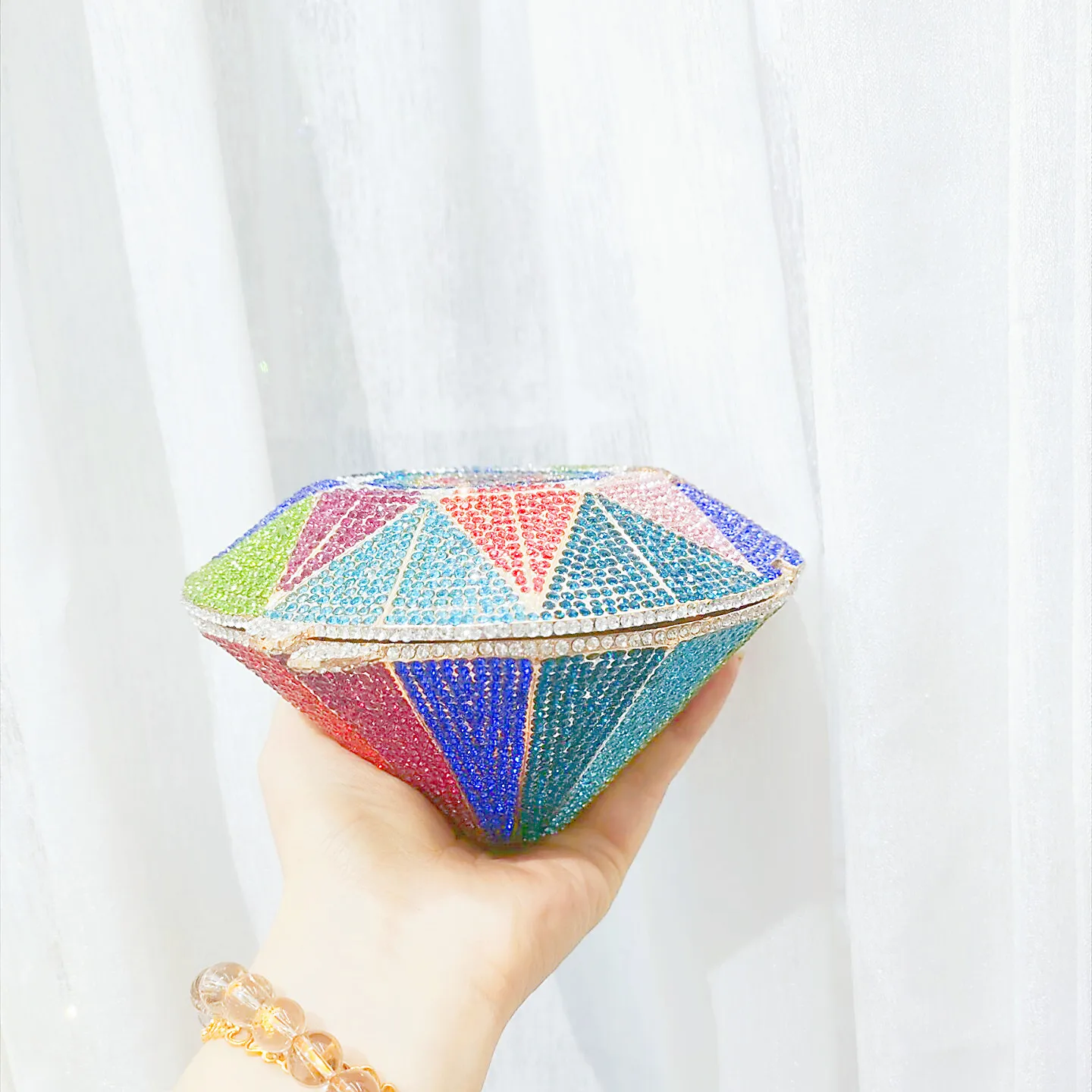A well-manicured woman's hand adorned with a gold beaded bracelet, featuring large, marble-sized beads in an orange hue, delicately holds an intricately adorned, diamond-shaped object against a backdrop of a sheer white curtain. This ornate accessory, reminiscent of a jewelry box, features a lid, suggesting it can open to secure items inside. The object is meticulously encrusted with glossy, shiny beads and tiny crystals in a vibrant array of colors, including dark blue, teal, light blue, red, magenta, lime green, light pink, purple, and orange. Each facet sparkles with elaborate beadwork, making it a captivating and colorful piece of art, beautifully contrasted by the simplicity of the white curtain and the elegance of the gold bracelet.